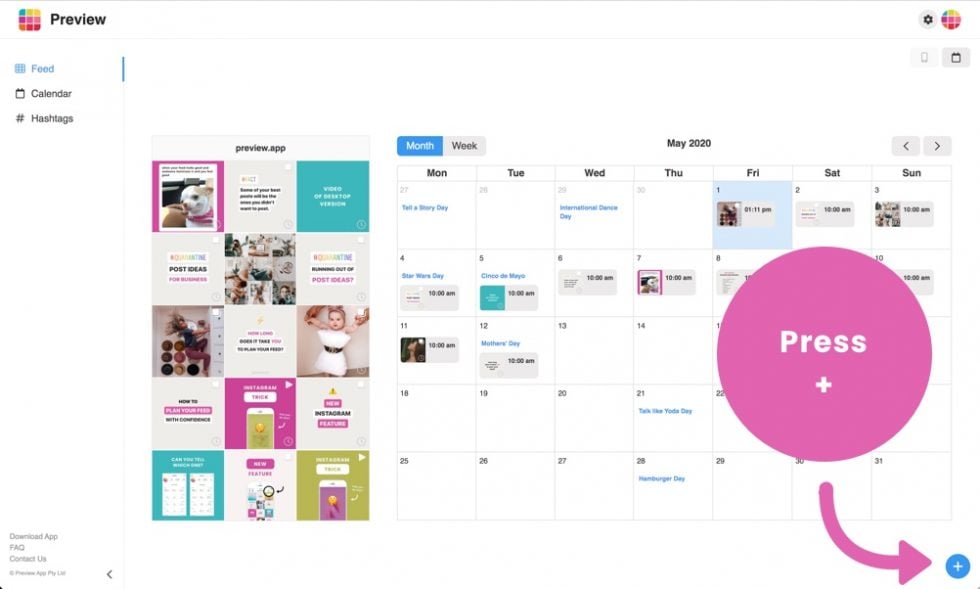This image depicts a highly detailed and colorful user interface layout, seen from a screenshot of an application. The primary background is light with a variety of colored elements organized across the screen.

In the top left corner, there is a small blue square followed by two yellow squares arranged horizontally. Directly below these squares is a sequence of dark purple, medium purple, and light purple squares. Further down, there are squares colored orange, red, and dark red, forming a larger square. To the right of this arrangement, the word "Preview" is displayed.

On the right side of the image, in alignment with the "Preview" label, there is a circle containing the same color configuration as mentioned earlier. To the left of this circle, there is a gray tab with a black settings icon.

Below the "Preview" label, entries labeled "Feed," "Calendar," and "Hashtags" are listed vertically in blue font, each accompanied by respective icons on their left side.

Towards the bottom, the interface displays links to "FAQ," "Contact Us," and "Download App."

About an inch below the top of the image, centrally positioned, is a black rectangular button with the text "Preview App" in bold. Adjacent to this button is a 3x5 grid of squares, totaling 15 squares, each containing various contents such as pictures and information.

To the right of this grid, a calendar is displayed. In the top left of the calendar, there is a blue tab with "Month" written in white and a gray tab with "Week" written in black. Centered at the top of the calendar, the text "May 2020" is visible. On the far right of the calendar, there are two gray square buttons, one featuring a right-facing arrow and the other a left-facing arrow.

The calendar layout includes columns labeled with the days of the week from Monday to Sunday. The month begins with May 1st on a Friday, and the 31st falls on a Sunday. Overlapping partially across the second, third, and fourth weeks of Friday, Saturday, and Sunday is a prominent purple circle with the word "Press" written in white inside it. Below this circle is a plus sign, followed by a thick purple arrow pointing downward and to the right.

In the bottom right corner of the image, there is a blue circle featuring a white plus sign.